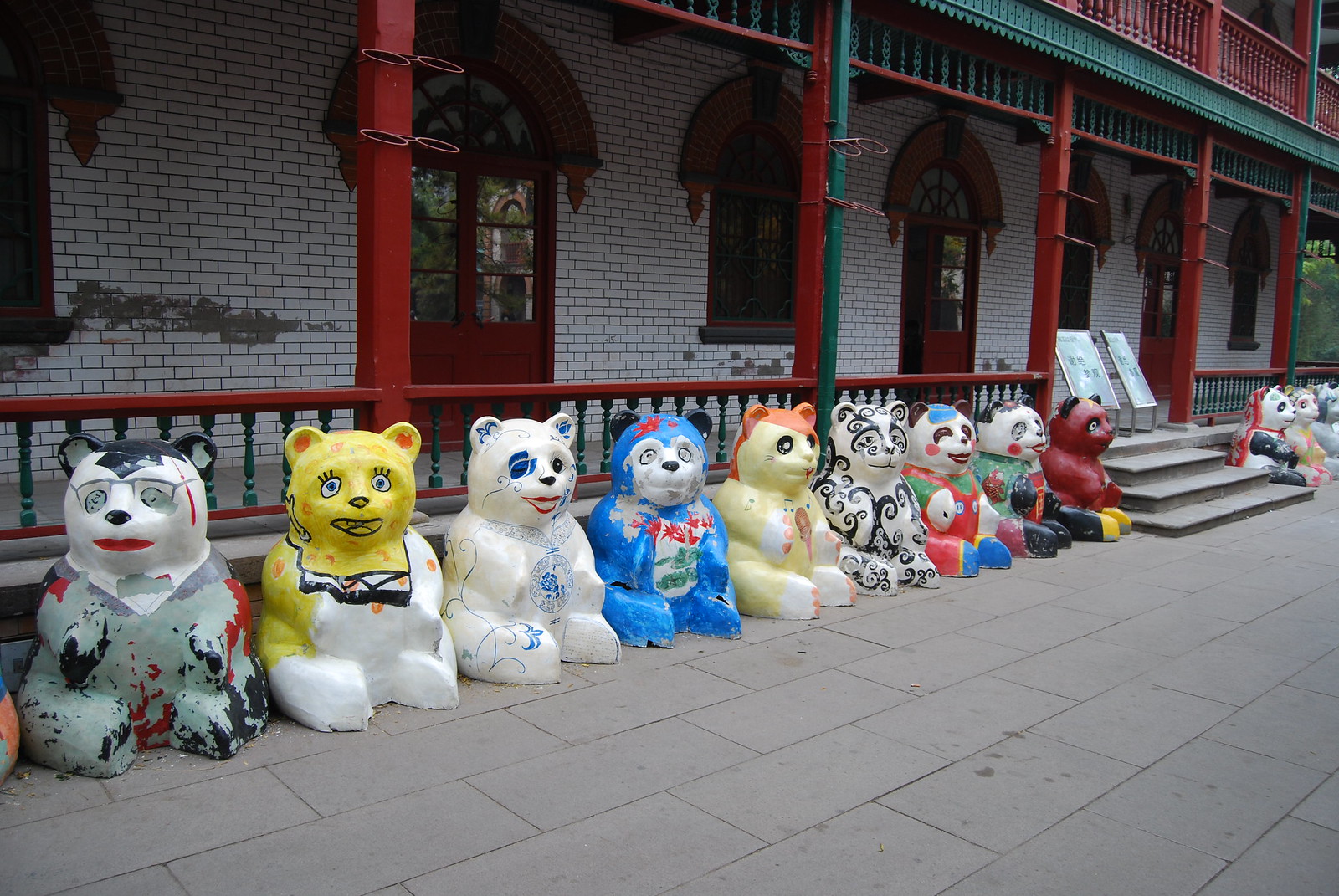The image showcases a striking building with distinct white brick or small white subway-shaped tiles, accented by deep red details on the window and door arches, festoon-type decorations, and red corbels. The structure features arched doorways and windows, supported by red posts that also sustain a visible portion of a second-story landing. This landing includes a railing with green details, creating a vibrant contrast. The photograph is cropped, revealing only part of the second story, leaving the building's full height unknown.

In front of this eclectic building is a spacious courtyard, paved with large, possible concrete tiles. The courtyard leads to the building via four broad, shallow steps without handrails. Flanking these steps and lining the edge of the courtyard are whimsical statues of teddy bears, each about three feet tall and crafted from what appears to be plaster or fiberglass. These bears are artistically painted, each bearing a unique design. Among the nine visible bears, one is dressed as a businessman with glasses and a suit, another is yellow with polka dots and eyelashes resembling a female bear, and others sport various imaginative patterns including floral designs and intricate black curlicues. More bears can be glimpsed past the steps, suggesting a larger collection. The overall scene hints at a cultural center or possibly a restaurant, given the elaborate decor and welcoming atmosphere.